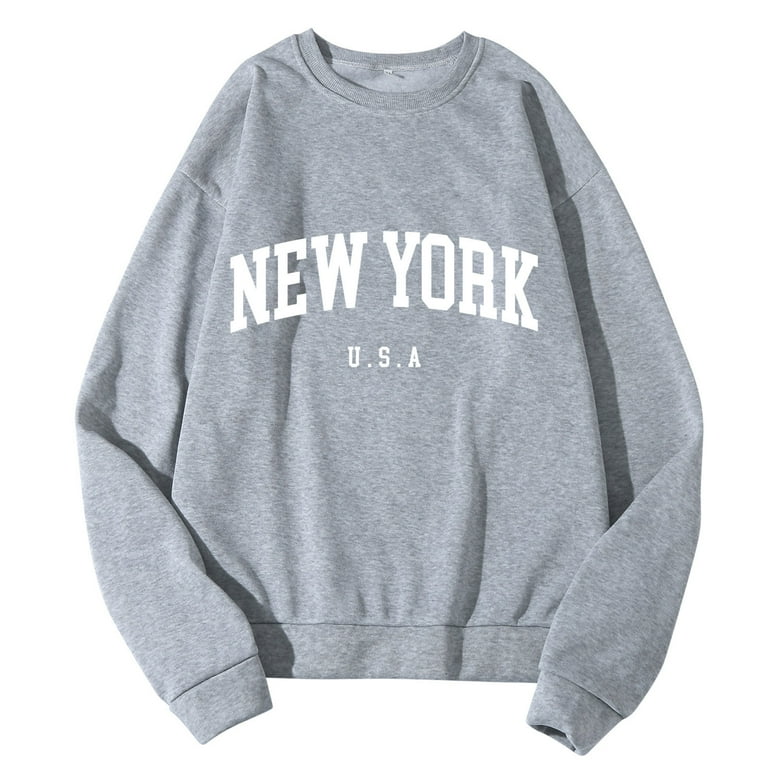The photograph showcases a gray, full-sleeved sweatshirt placed on a white background. The sweatshirt features bold, capitalized text "NEW YORK" prominently displayed across the chest in an arch-like fashion, with "USA" written below in a smaller font. The text is white, providing a striking contrast against the gray fabric. The sweatshirt, which appears to be a simple cotton material and potentially styled for females, includes detailing such as tapering at the wrists and waist, as well as stitching at the neckline. The casual, round-neck design and absence of a visible label underscore its simple, yet fashionable appeal. The overall theme of the image emphasizes casual apparel with a focus on fashion and comfort.